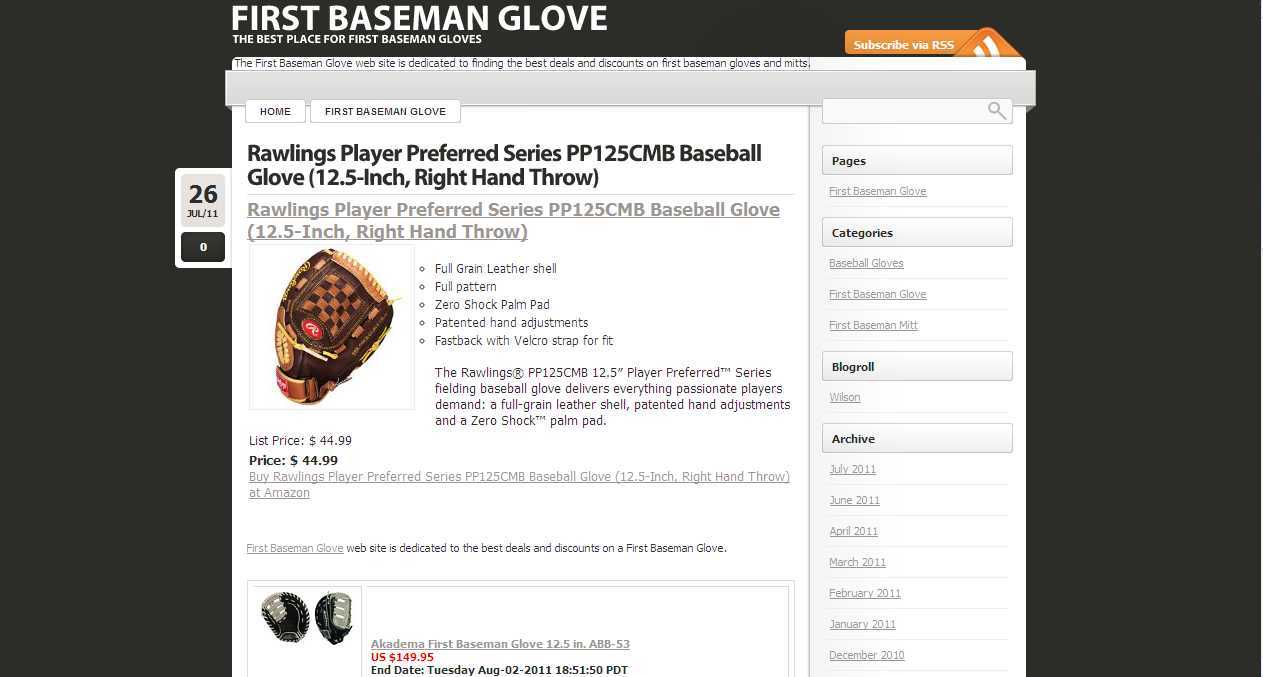The image is a screen capture of a dated e-commerce website with a black background and a white browser interface, accompanied by a sidebar for navigation. The site prominently displays a header image that promotes first baseman gloves with the tagline, "First Baseman Glove, the best place for first baseman gloves," in a basic white font resembling Helvetica or Arial. Below this header, the main content features a detailed product listing for a "Rawlings Player Preferred Series PP125CMB Baseball Glove" in brackets, specifying it as a 12.5-inch right-hand throw glove. The detailed description includes features such as a full-grain leather shell, full pattern, zero shock palm pad, patented hand adjustments, and a fast-back with a velcro strap. An image of the brown baseball glove with dark brown checkering is also displayed. The price of the glove is listed at $44.99. Adjacent to the product description, there's a sidebar displaying additional navigation options, a search bar, and a list of recommended products, one of which is priced at $149.95. A timestamp indicating "final date Tuesday, August 2nd, 2011 at 18:51:50 PDT" is noted, adding to the overall dated appearance of the website. The layout is fairly generic, with a gray two-column template and a simple white logo. There's also a button at the very top of the page labeled "subscribe via RSS."